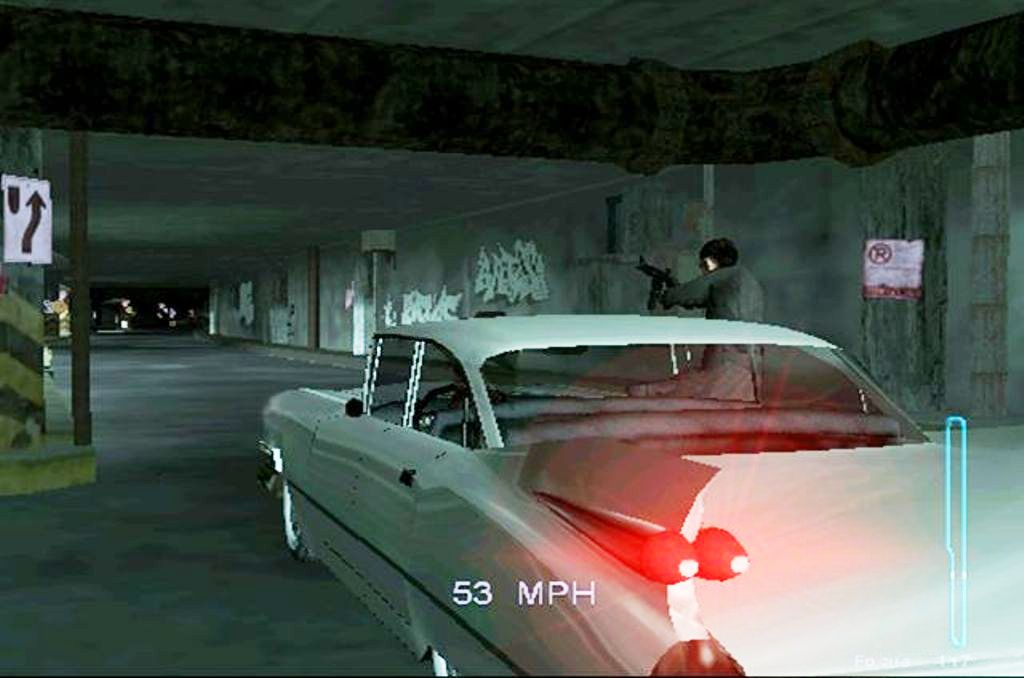The image is a screenshot from an old or retro-styled video game, depicted in a landscape orientation and somewhat pixelated. At the center of the image, a white, old-style Mustang car is seen driving into a parking garage. The car’s back end is facing the bottom right of the image, with a person leaning out of the passenger window holding a long-neck machine gun. This individual is dressed in a hat, a grey sweatshirt-type jacket, and pants.

The setting is an old, worn-down parking garage with graffiti on the tunnel walls. Above, thick brown pipes run along the concrete ceiling. A sign to the left reads "This way around an island," below which black and yellow vertical stripes are visible. The garage opens at the far end, allowing light to filter through. At the bottom of the screen, white font displays "53 MPH," and the bottom right features a slender blue outline, perhaps indicating a track. The overall image quality is low, and the driver of the car is not visible. Additionally, the back of the car shows an object resembling a rocket ship, and a "No Parking" sign is also present in the scene.